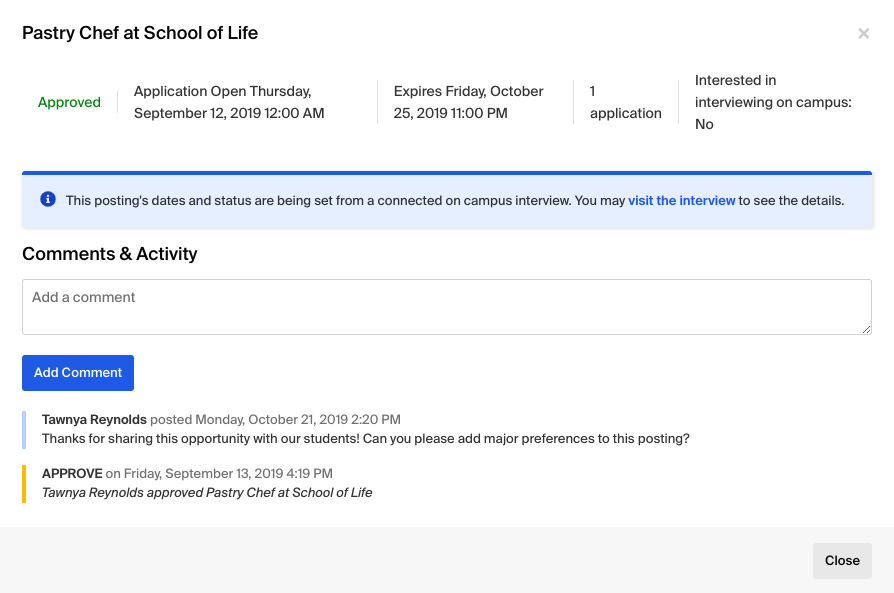**Detailed Caption:**

This image showcases a school website dedicated to culinary arts education, specifically highlighting an announcement for a Pastry Chef program. On the left side of the screen, a green label marks the program as "Approved." The application period is prominently displayed, beginning on Thursday, September 12 and running until Friday, October 20, 2019, with specific times listed (until 12 a.m. on September 19 and 11 p.m. on October 20).

The announcement seeks to inform students that no on-campus interviews are required for the application. Additionally, there is a blue informational tag with black text, providing further details and a hyperlink in light blue text labeled “visit the interview” for more information.

Below the main announcement, there is an interactive section where users can leave comments or activity notes. Currently, there are no comments, and a blue bar with white text encourages users to “add a comment.”

A comment from user Tyra Reynolds, dated Monday, October 21, 2019, at 2:20 p.m., is displayed. Tyra thanks the administration for sharing the opportunity with students and requests the addition of major preferences to the posting. The post also notes that the Pastry Chef program was approved on Friday, September 13, 2019, by Tyra.

At the bottom right of the screen, there is a "Close" option, and the website seems to be part of a messaging system tailored for baking or culinary schools, indicating the successful approval of the application related to the Pastry Chef program.